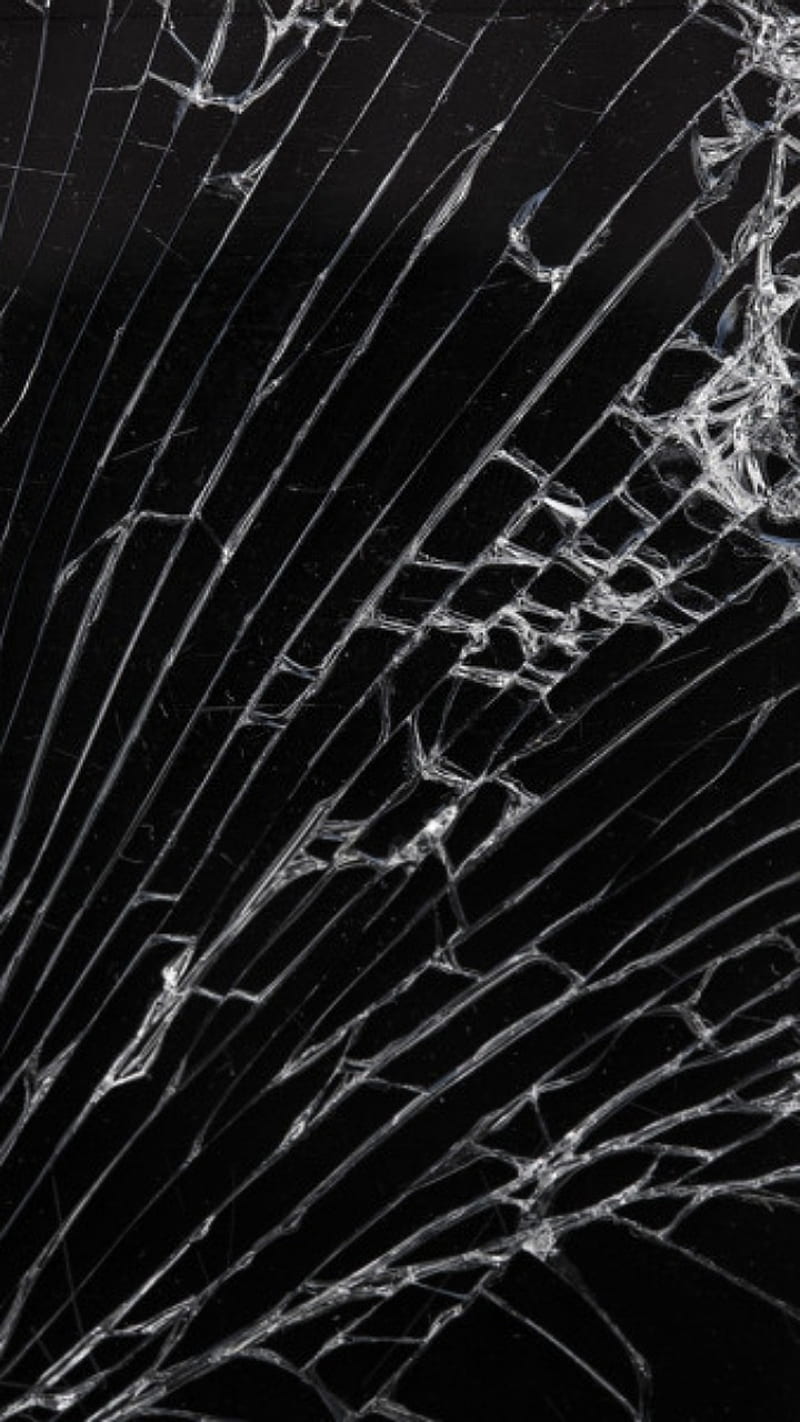A detailed close-up image showcases an intricate network of spider webs set against a black background. The spider webs originate predominantly from the bottom left corner, where the lines converge more closely together. Radiating outward, there are at least 26 notable strands, some of which cross over each other, creating thicker patterns especially in the central region. The central section also features lines that intertwine, appearing as if they are composed of three or four combined strands. Just above the right center edge, there's a triangular formation pointing leftwards, which seems to be housing a wrapped-up bug or a creature. The fine, silky lines resemble the delicate fractures of shattered glass, giving the impression of a glass plane cracked in a spider-man-like circular pattern. Some of these lines extend straight outwards, most notably towards the upper center area, further adding to the complexity and beauty of the scene.